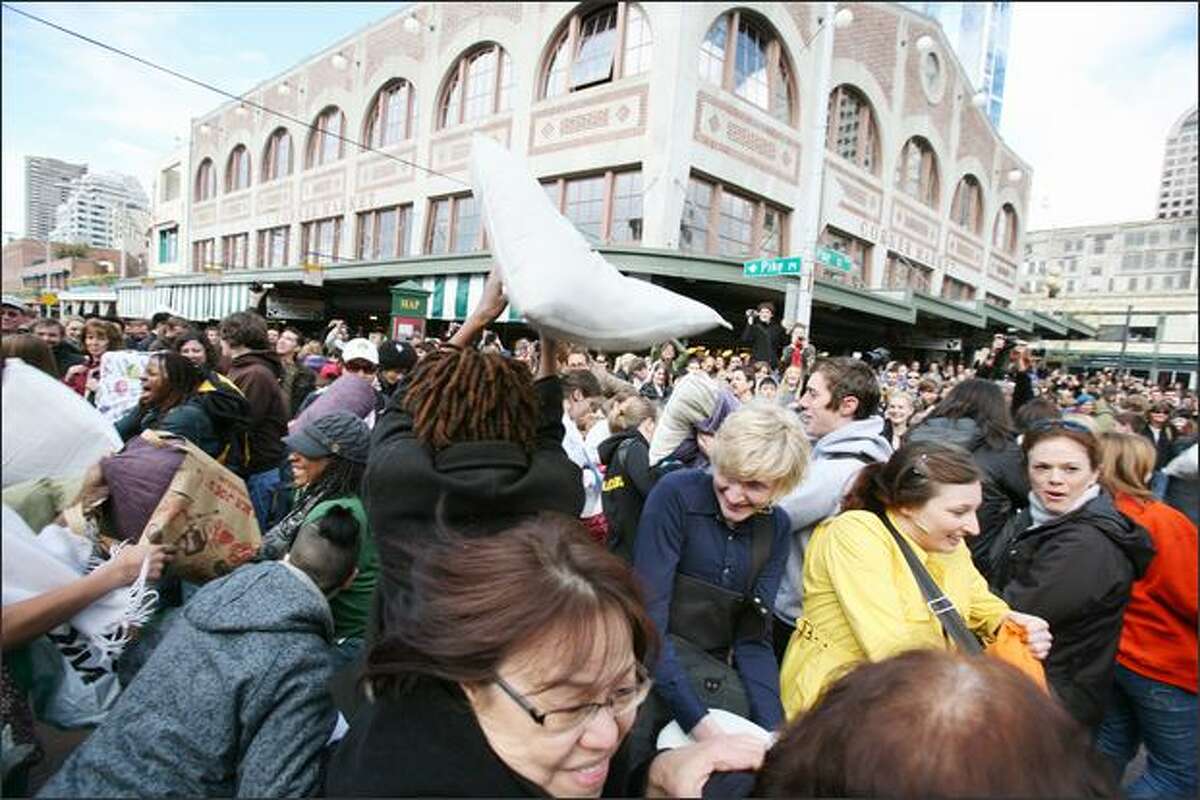A vibrant street scene in a bustling city captures a large, joyful crowd filling the road. The foreground is packed with people laughing, smiling, and holding bags, goods, and food, leaving little room to walk. Their clothing spans a spectrum of colors, including yellow, dark blue, orange, red, black, green, pink, and purple. Behind them, a prominent building showcases two-story windows with arched frames on the top floor, while additional buildings can be seen on either side. Street signs, including one that may read "Pine," punctuate the background, adding to the urban ambiance. The sky is a clear blue with scattered clouds, and the bright sunlight enhances the cream and brown hues of the buildings. This scene could depict a lively event or gathering, capturing the essence of communal enjoyment in a major city.